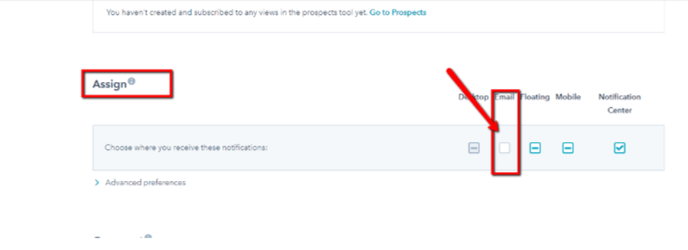The image displays a user interface with a primary message stating, "You haven't created and subscribed to any views in the prospects yet. Go to prospects." The message is highlighted in blue.

Below this message, there is a prominent red button labeled "Sign," enclosed in a red-bordered box.

A section underneath offers notification preferences in a gray box. The options available are: Desktop, Email, Floating, Mobile, and Notification Center, all aligned in a single row.

- Desktop: Has a blue minus sign within a square.
- Email: Marked by a red arrow pointing diagonally downward from the top right, enclosed in a red box, and currently not selected.
- Floating: Displays a blue minus sign within a square.
- Mobile: Features a blue minus sign within a square.
- Notification Center: Indicated by a blue checkmark.

Toward the bottom left corner, there is a blue arrow pointing to "Advanced Preferences."

The entire interface has a white background with black text. Additionally, there is a small floating element encased in a red-bordered circle beside the email option, which likely indicates additional notification settings related to emails, highlighted by a vertical box including the white part of this section.